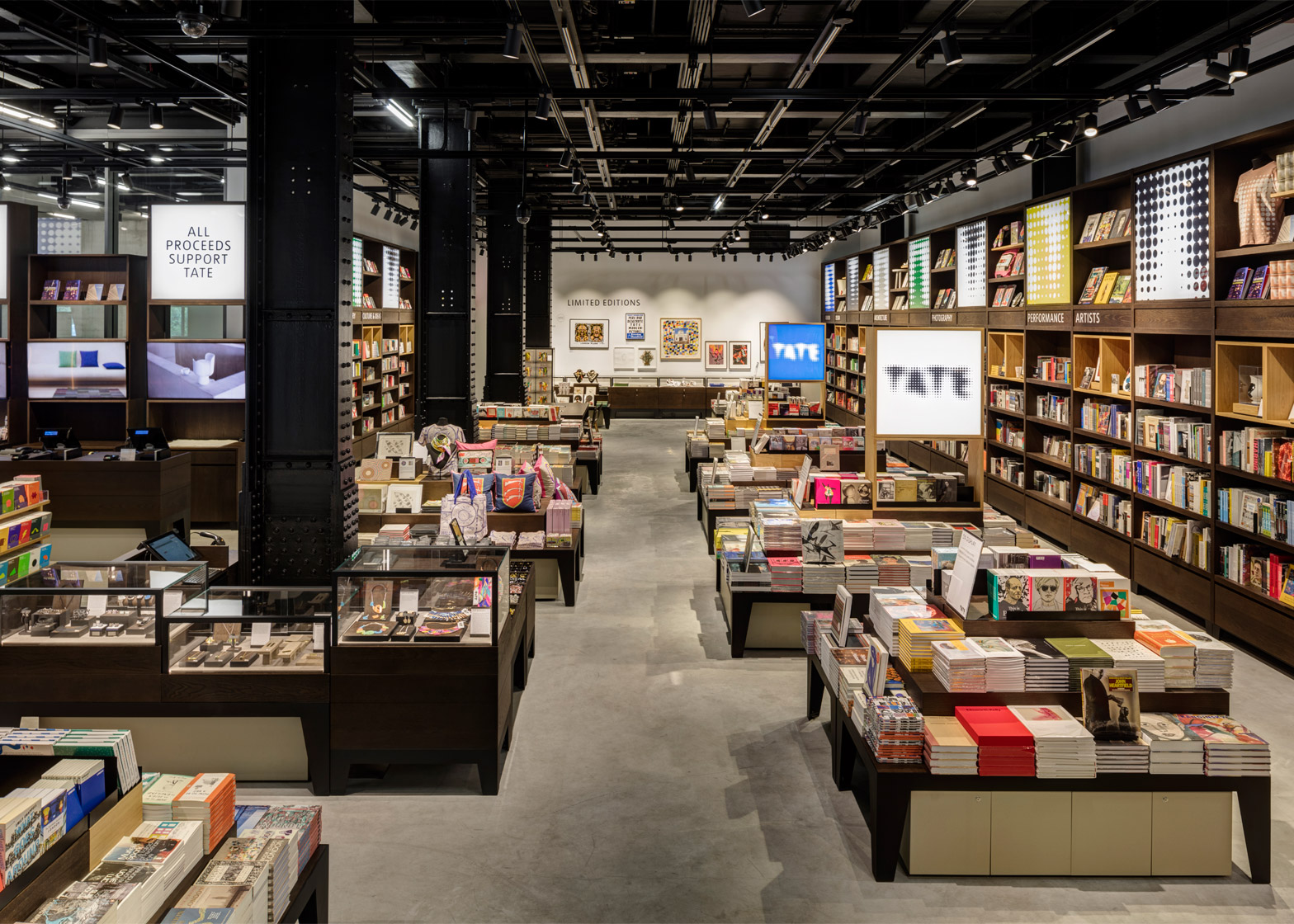This photograph captures the interior of a large warehouse-turned-store, bustling with items for sale. The expansive space features a gray concrete floor and an open ceiling with black metallic structures, including crisscrossing horizontal and vertical bars. The ceiling also displays a network of pipes. Along the right side of the store, brown shelving units house an extensive collection of books. Positioned in the middle, large square tables stacked with more books dominate the floor space. To the left, glass-encased displays showcase a variety of jewelry items. Supporting the roof are tall black metal columns, one of which bears a sign reading "All Proceeds Support Tate." The front wall, painted white, is adorned with various artworks, illuminated by ceiling lights. The same white wall features additional paintings, enhancing the creative ambiance of the store. Notably, other miscellaneous items are scattered throughout, adding to the diverse shopping experience.